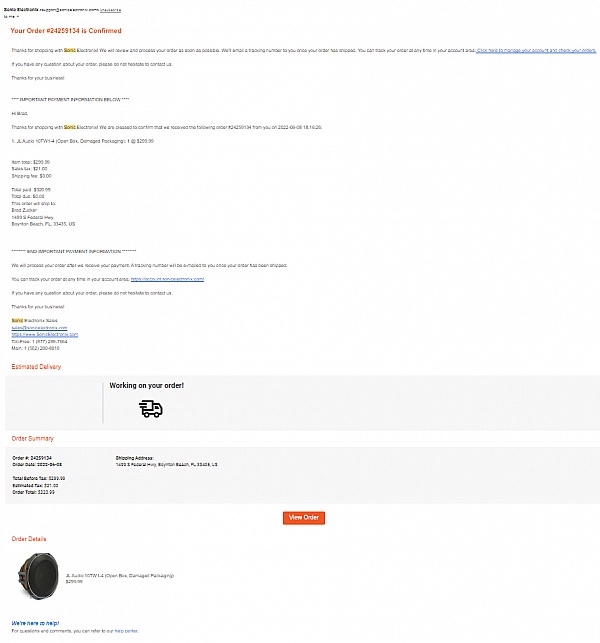This is an invoice or order confirmation screenshot. At the top, written in bold orange text, it states: "Your order number 24259134 is confirmed." Beneath this header, there's grey text that is blurred, with the fifth word highlighted in yellow. On the right side of this line, underlined in blue, is the text that starts: "Click here to manage your account and check your orders." Following this, there are two more lines of text.

Next, centered within a line of asterisks, it reads: "Important pick-up information below." Beneath this notice, there are three lines of text, with the second line also having its fifth word highlighted in yellow. Following this section are three lines of grey text detailing information alongside some dollar amounts. Below this, there are six additional lines of grey text that are too blurry to decipher.

Highlighted by another line of asterisks is the text: "End important payment information." Below this, there are four more lines of grey text. 

At the bottom of the page, an orange line of text reads: "Estimated delivery." Beneath this, a black clipart image of a truck is accompanied by the text: "Working on your order." Following this, in orange text, it states: "Order summary," with legible black text appearing below it within a grey box. Finally, at the bottom, there's an orange button featuring white text that says: "View order."